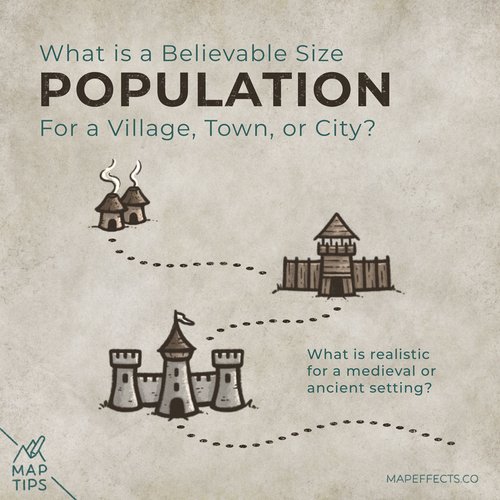The image is a simplified instructional map on a grey-beige background, illustrating the concept of population sizes for different types of medieval or ancient settlements. At the top, text reads "What is a believable size" in green letters, followed by "population for a village, town, or city?" in black and green letters. The map includes small drawings on the left: two tiny brown huts with straw roofs, chimney smoke, and arch doors. A dotted line connects these huts to a slightly larger wooden home with a pointed roof, indicating progression. Further along the dotted line, the map depicts a medieval castle with a flag atop its central tower. Additional text states "What is realistic for a medieval or ancient setting," and labels like "map tips" and "map effects" are present, suggesting educational or reference purposes.